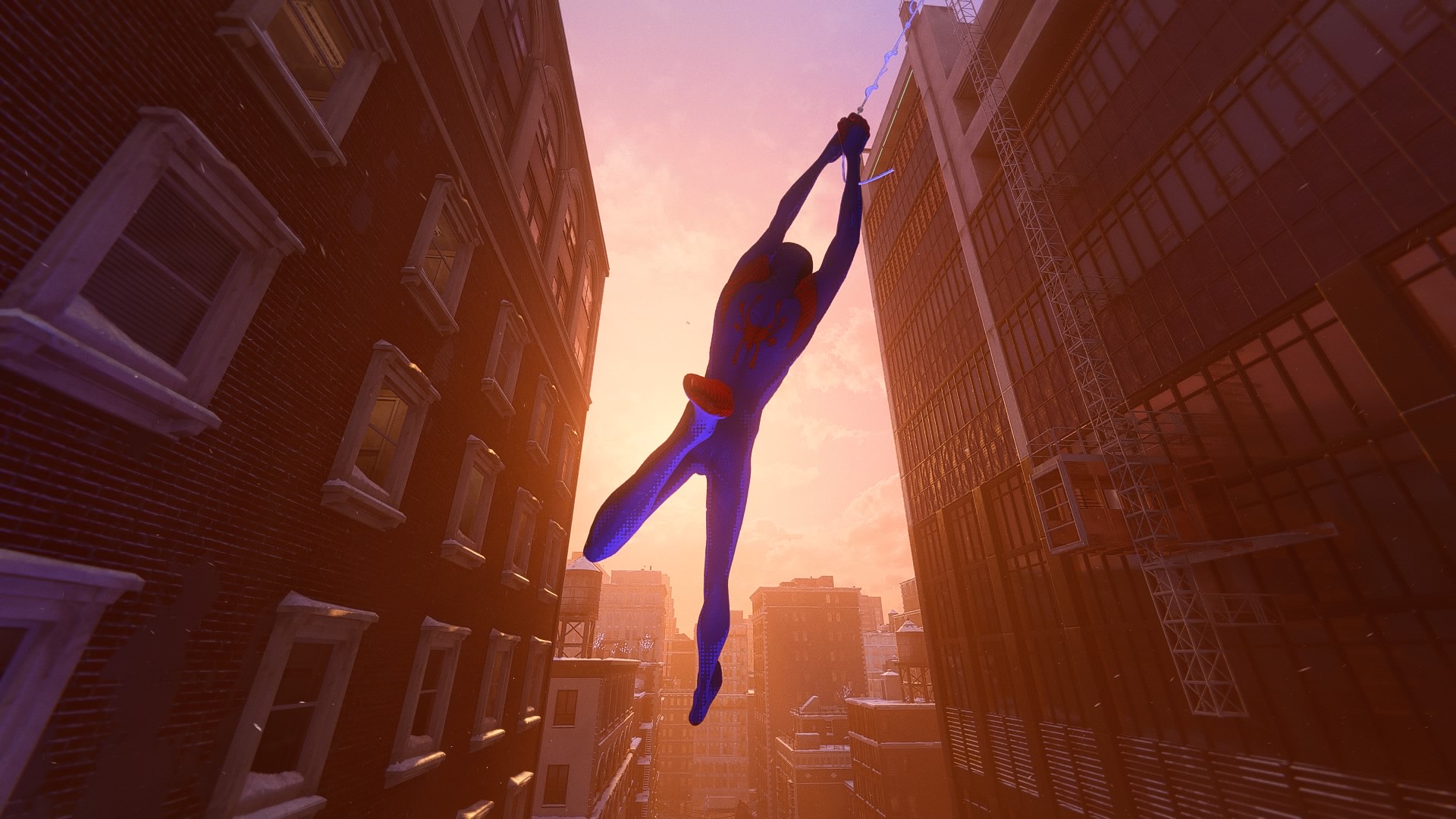In this detailed cityscape, a close view reveals towering buildings with numerous windows reflecting light, adding a dynamic texture to the scene. Dominating the center, Spider-Man is in mid-swing between two prominent buildings that are close to each other. Wearing his iconic red and blue suit, highlighted by red boots, spider motifs on his shoulders and chest, and red accents up his legs, Spider-Man's vibrant colors stand out against the backdrop. He is clinging to a silvery web thread, stretched out vertically and leaning slightly to the right. The sky above transitions from a golden-light yellow to a light purple, dotted with clouds, creating a dramatic and vibrant horizon. The sun shines brilliantly between the tops of the two buildings, framing Spider-Man's acrobatic form. On the left, a brick building features four rows of white square windows, while the right building, with its warehouse-like appearance, has large, expansive windows and a white metal antenna tower rising alongside it. Beyond, the cityscape continues with more tall buildings, completing this striking and dynamic urban scene.